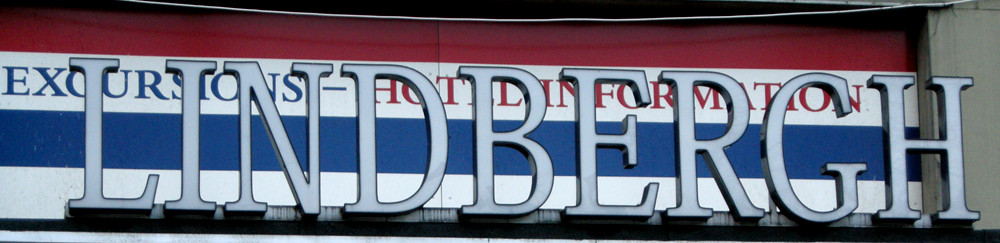The image features a white sign with the word "Lindbergh" in a basic, unadorned font. The sign appears to be backlit, suggesting it illuminates at night. Behind this sign, partial text can be seen, referencing "Excursions" and "Hotel Information." The word "Excursions" is in all capital letters and blue, while the phrase "Hotel Information" follows in red, both in the same plain font as "Lindbergh." Above this text is a red stripe, and the background where "Excursions, Hotel Information" is written is a white stripe. Below this section is another stripe, this time in blue. The overall design is minimalistic, but the color-coding and backlighting indicate a functional and informative sign, likely aimed at tourists or guests.